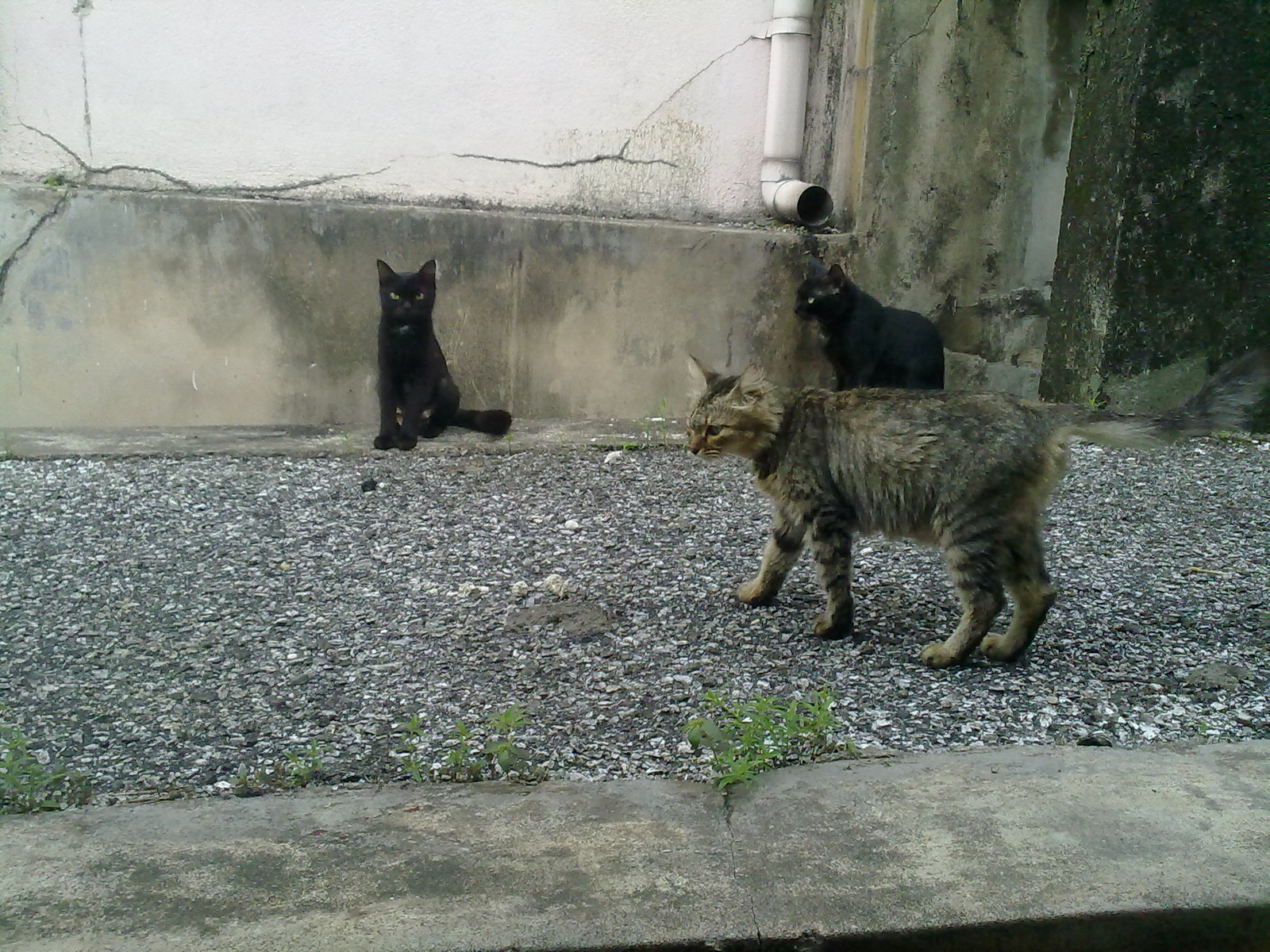In this colorful, landscape-oriented photograph, a gritty urban scene unfolds. The backdrop features a grimy, grayish-white concrete wall, streaked with mold and algae, accentuated by a white drain pipe stretching down from the top middle. The ground in the foreground consists of crushed stones interspersed with patches of weeds and a narrow strip of pavement.

Three cats, each distinct in its appearance and positioning, inhabit this space. Alongside the wall, closest to the background, a skinny, homeless-looking black cat sits solemnly, its dark fur contrasting sharply against the dirty wall. Another black cat stands at the edge of the building, gazing directly into the camera, its body oriented towards the other black feline. At the forefront, a well-fed striped brown tabby cat strides purposefully across the rocky ground, its grayish-brown fur blending with the earth tones of the surroundings. The tabby, slightly right of center, faces towards the left, adding a dynamic element to the otherwise still scene.